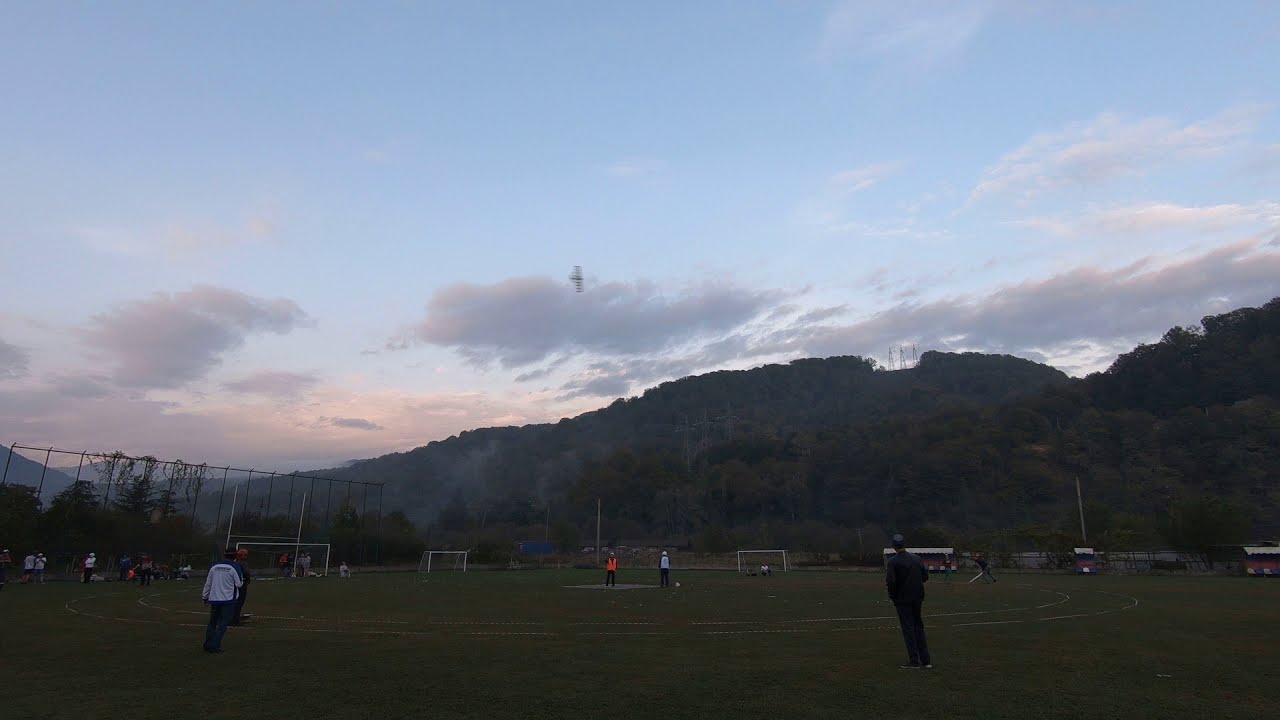The image depicts a verdant soccer field framed by mountains in the background, under a sky painted by the hues of a setting or rising sun. A group of adults is gathered on the grassy expanse, with some standing towards the left side and others near the middle, seemingly engaged in an activities like attempting to land a helicopter or observing something in the air. The man on the right sports a black shirt, joined by another similarly dressed individual in dark pants on the left. A sizeable fence runs along the left side of the field, beyond which some spectators are visible, and a few buildings dot the right-hand side of the scene. The field is lush and green, accentuated by a scattering of soccer nets, and the overall atmosphere suggests an impending dusk, with the low clouds accentuating the tranquil yet lively setting.